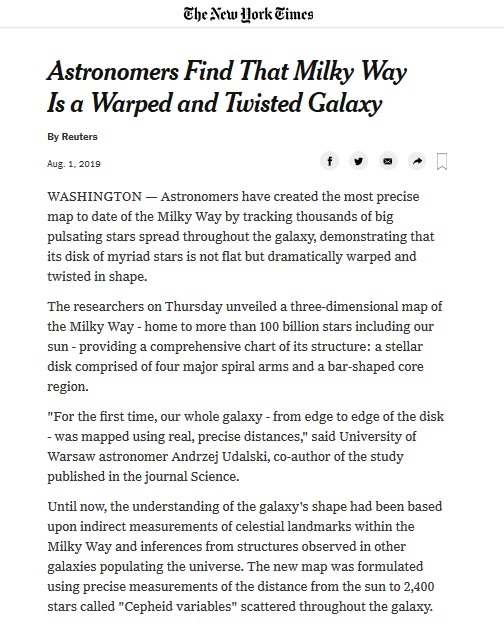A detailed image caption based on the provided voice description might look like this:

---

"Image with white background featuring an article from The New York Times. The headline reads, 'Astronomers find that Milky Way is a warped and twisted galaxy,' published by Reuters on August 1, 2019. The image includes social media icons for Facebook, Twitter, an envelope symbol, a thought bubble resembling a 'Reply' function, and a bookmark icon. The article's excerpt begins with 'Washington – Astronomers have created the most precise map to date of the Milky Way by tracking thousands of pulsating stars spread throughout the galaxy, demonstrating that its disk of myriad stars is not flat but dramatically warped and twisted in shape.' On Thursday, researchers unveiled a three-dimensional map of the Milky Way, which is home to more than 100 billion stars including our Sun. This map provides a comprehensive chart of its structure, highlighting a stellar disk comprised of four major spiral arms and a bar-shaped core region."

---